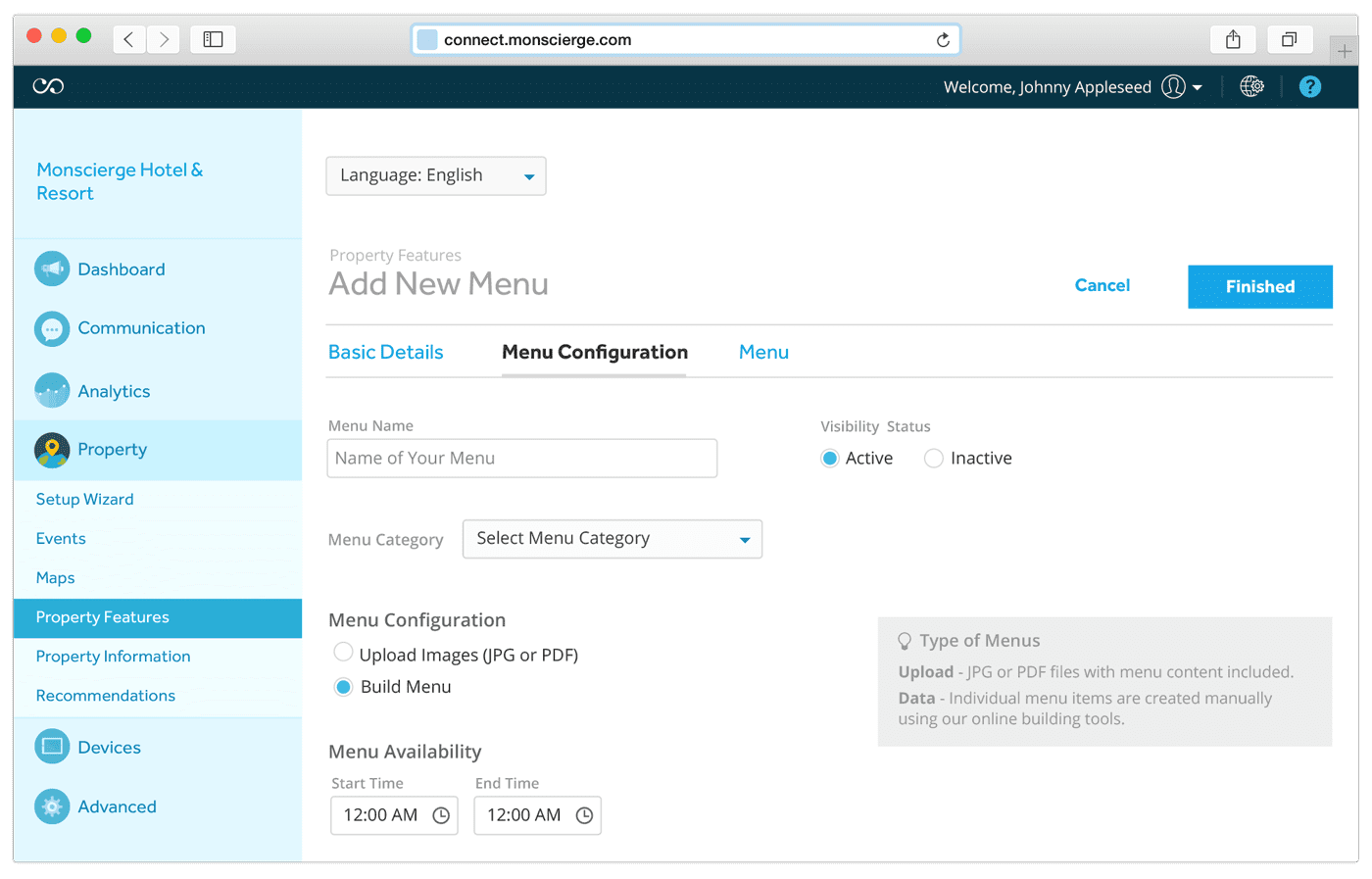This detailed caption provides a comprehensive overview of a screenshot taken of a desktop or laptop computer, which appears to be a Mac, displaying a web browser opened to the website connect.moncierge.com.

---

This screenshot captures a detailed view of a desktop or laptop computer, presumably a Mac, displaying the web browser opened to connect.moncierge.com. At the top of the screen, there's a dark green banner featuring a welcome message for "Johnny Appleseed," accompanied by a help button and an account button. 

On the left side of the screenshot, there's a sidebar labeled "Montierge Hotel and Resort," which includes various navigation buttons such as Dashboard, Communications, Analytics, Property, Setup Wizard, Events, Maps, Property Features, Property Information, Recommendations, Devices, and Advanced. 

To the right, the main content area features a drop-down menu for selecting a language, with English currently chosen. Below this drop-down, the title "Property Features" appears within a new menu interface. There are also Cancel and Finish buttons situated on the right side of the screen.

In the main content section, several elements are outlined, including Basic Details, Menu Configuration, and Menu Sections, with Menu Configuration currently selected. The Menu Configuration screen includes fields for entering the menu name, setting visibility status, and selecting a menu category from a drop-down list. Additional configurable options include menu availability, with drop-downs to set start and end times, as well as a tips section that details the different types of menus and explains the distinctions between upload and data.